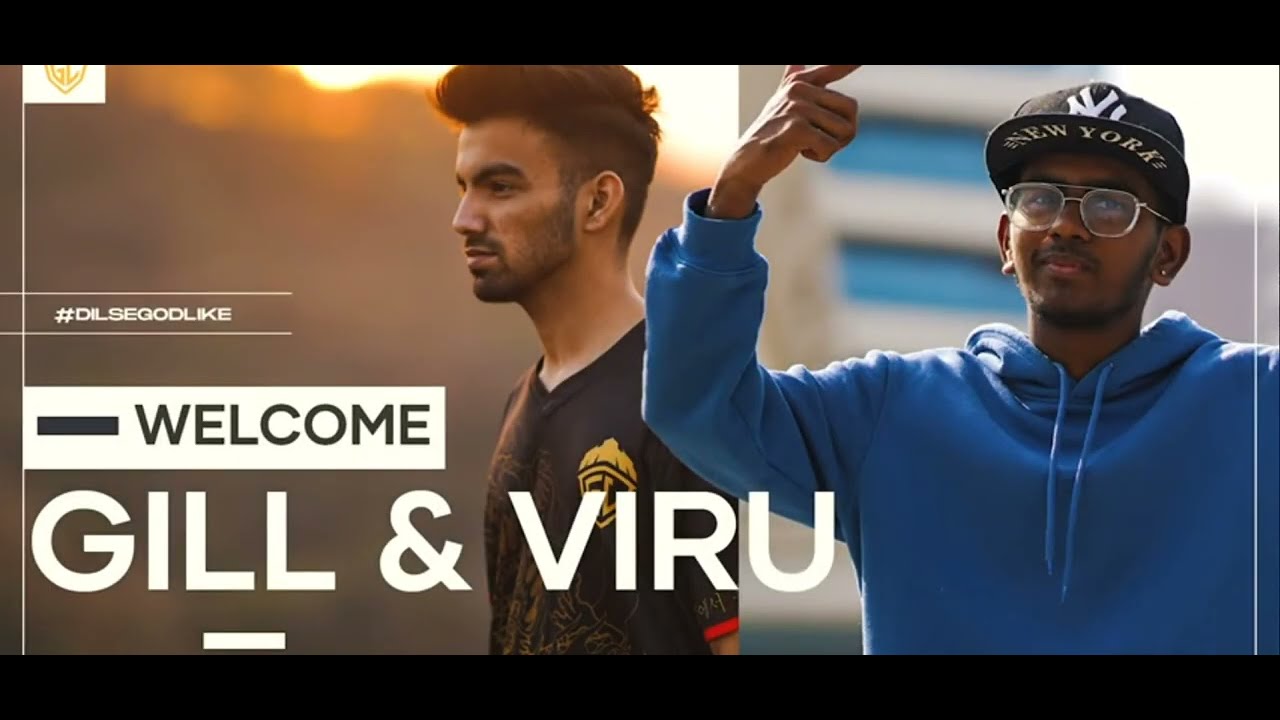The image is a promotional, landscape-oriented color photograph featuring two young men against distinct backgrounds, separated by a black stripe at the top and bottom. On the left side of the image is a man with a darker complexion, medium-length puffed up hair, wearing a black v-neck shirt with red trim and a gold emblem on his chest. He sports a moustache and beard, and appears to be walking outdoors during sunset, with a mountain and sky visible in the background. On the right, a darker-skinned Indian man stands, aged around 16-18 years, wearing a blue hoodie and a black Yankees cap with "New York" written on the underside of the brim. He has glasses, an earring, and gestures upwards with his right hand, set against a daytime backdrop featuring a tall white or silver reflective building. Overlaid in the middle of the image is the handle "#DILSEGODLIKE" above a white bar with the label "WELCOME" and the names "GIL & VIRU" in bold, white, sans-serif text. The top left corner includes a logo featuring the letters "GC" in gold on a white shield.